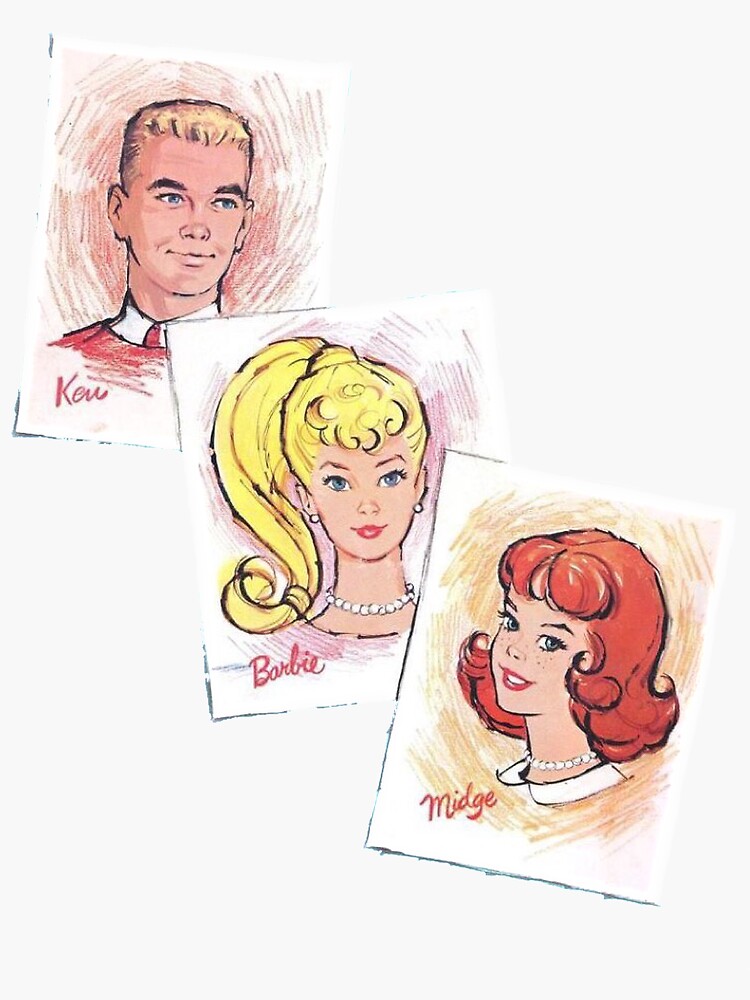The image features detailed, cartoon-like sketches of three classic Barbie characters, with each character depicted in individual, overlapping squares resembling vintage headshots. In the top left, Ken, with short blonde hair, wears a red shirt with a distinctive white collar. The background behind him has a reddish hue, and his name "Ken" is inscribed in the bottom left of his square. In the center, we see Barbie, who flaunts her iconic long blonde hair, bright blue eyes, and a white pearl necklace. The background here is textured in pink, adding a signature touch to her appearance, while her name adorns the bottom of her image. To the bottom right is Midge, characterized by her red hair and white pearl necklace. She wears a white Peter Pan-like collar on her shirt, and the background is textured in orange. Her sketch is labeled "Midge" in the bottom left corner. All three images are artistically drawn with vibrant colors and seem to be created using colored pencils or markers. The arrangement of the squares gives the impression of a nostalgic photograph collage.